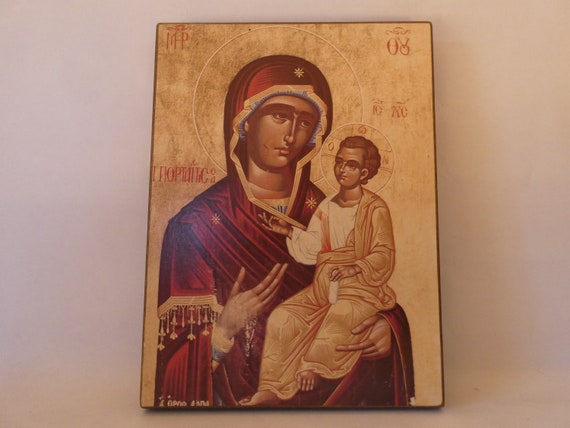The detailed image is a photograph of a painting of the Madonna and Child mounted on a pink wall, with the painting framed by a thin brown border. The background of the painting is a golden hue, adorned with red Greek text that's not legible. The Madonna, positioned on the left, is portrayed with tanned skin and draped in a flowing red robe adorned with gold decorations, including a small star above her head. She gazes downwards, holding the Christ Child in her left arm. The Child, depicted as mature-looking, wears a golden robe over a white shirt, with one foot bare. He looks up at the Madonna with a halo around his head, mirroring the halo around hers. The composition is softly illuminated from the left side, casting a shadow on the painting's right side, and the textured background features beige and brown tones.